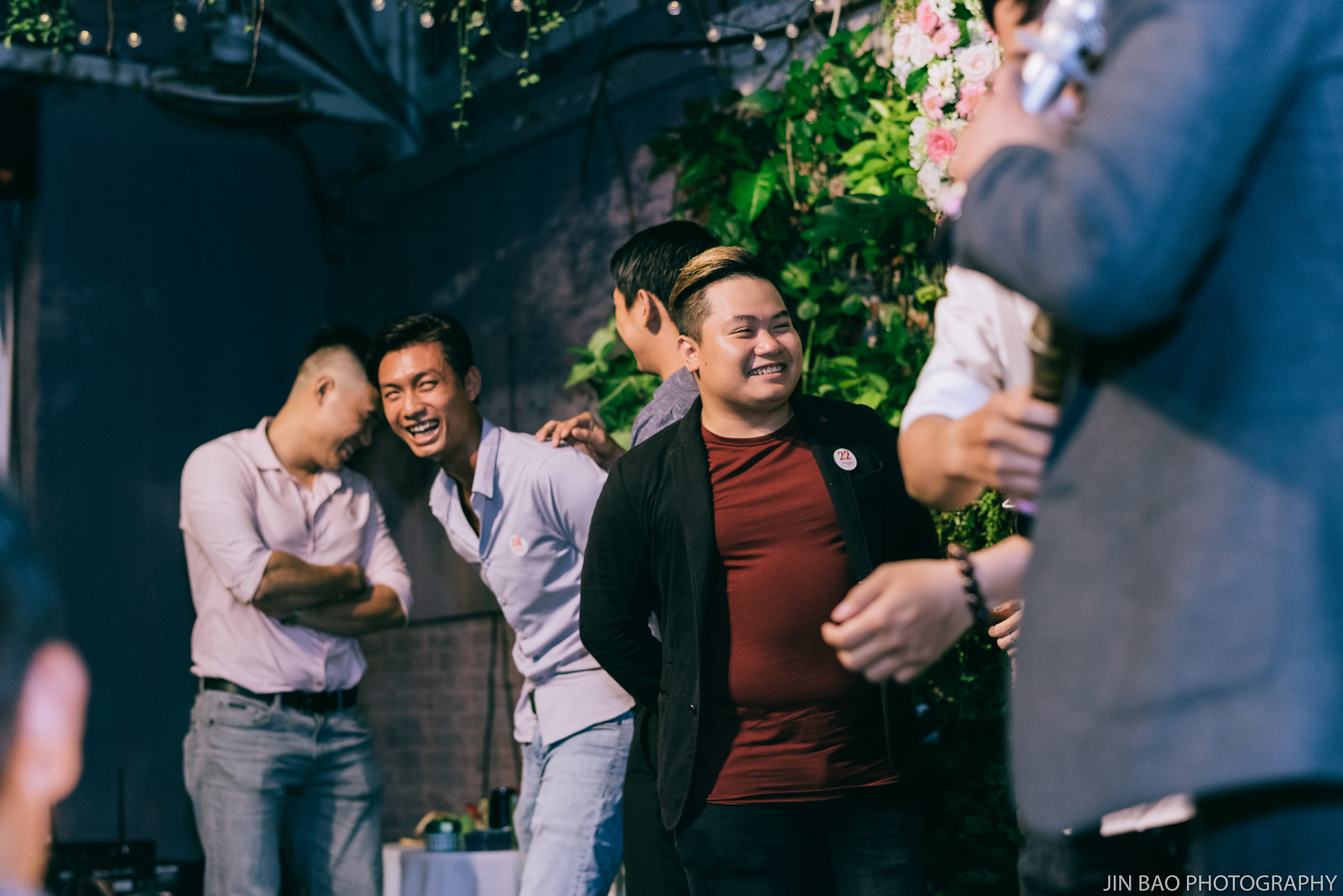The image, taken by Jin Bao Photography, depicts a lively social event, possibly outdoors or in a patio area adorned with green foliage and decorative lighting hanging from above. At the center of this landscape-oriented color photograph, four men are engaged in animated interaction. On the left, a man in a light gray shirt with sleeves rolled up to his elbows, gray trousers, and a belt stands with his arms folded, looking down and to his side. Next to him, another man with black hair is leaning forward towards the camera, smiling, wearing a blue shirt and jeans. To his right, a third man is visible by the side of his head, which is turned towards the second man. The fourth person is heavier set, with distinctive black and blonde hair shaved short at the sides. He is smiling and looking up to the top right corner, dressed in a T-shirt and a black blazer with a badge on it. The two men on the far right are blurred, holding microphones, and partially out of the frame. The background features vibrant greenery, flowers, and party lights that add to the festive atmosphere, creating a vivid representation of the joyful gathering.